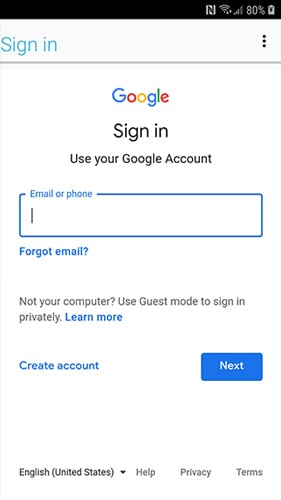The screenshot depicts the sign-in page for Google's online services on a smartphone. At the top right corner of the screen, several status icons are visible, including the battery percentage and Wi-Fi signal. Below these icons, on the left side, there is a blue text link labeled "Sign in."

Centered on the page is the colorful Google logo, followed by the phrase "Sign in" in black text, which is not a clickable link. Below this, the instruction "Use your Google Account" is displayed.

Underneath the instructions, there is a text box outlined in blue, with the placeholder text "Email or phone" also in blue. Directly below this, there's a blue link stating "Forgot email?"

The next section provides the option to use guest mode for private sign-in with the text, "Not your computer? Use Guest mode to sign in privately." Following this message, there is another blue link labeled "Learn more."

Further down, there is the option to "Create account" shown in blue text. On the same line, towards the right, a blue button with white text reads "Next."

At the very bottom of the screen, there are four menu options. The first is a dropdown menu labeled "English (United States)," followed by three links: "Help," "Privacy," and "Terms."